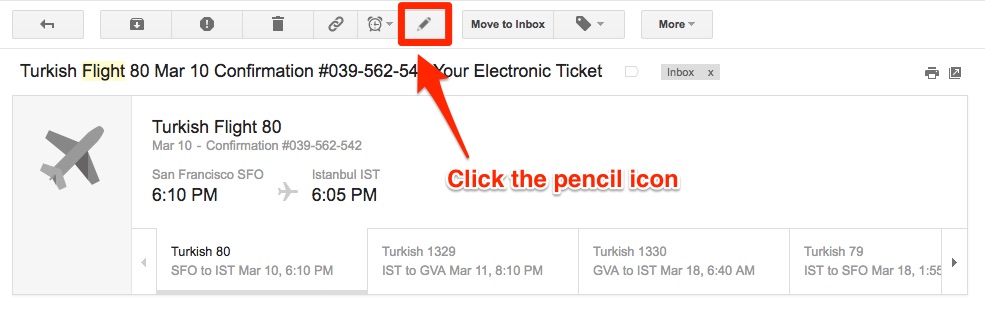The image depicts a section of a web page with a stark white background. At the top of the page, there is a horizontal menu bar housing various action buttons. From left to right, the buttons include:

1. A back arrow icon
2. A folder icon
3. A stop sign icon featuring an exclamation point
4. A trash can icon
5. A link icon
6. A clock icon
7. A pencil icon surrounded by a bold red outline
8. A "Move to Inbox" option
9. A price tag icon
10. A drop-down box labeled "More."

Additionally, a large arrow is pointing towards the highlighted pencil icon, accompanied by the text "Click the pencil icon," suggesting a specific action to be performed.

Below this instructional banner, the web page displays detailed flight information for a Turkish Airlines reservation, including confirmation numbers, electronic ticket details, and flight times both for departure and arrival at various locations. The page seems to serve as a guide, instructing the user on the necessary steps to manage or amend their flight reservation.